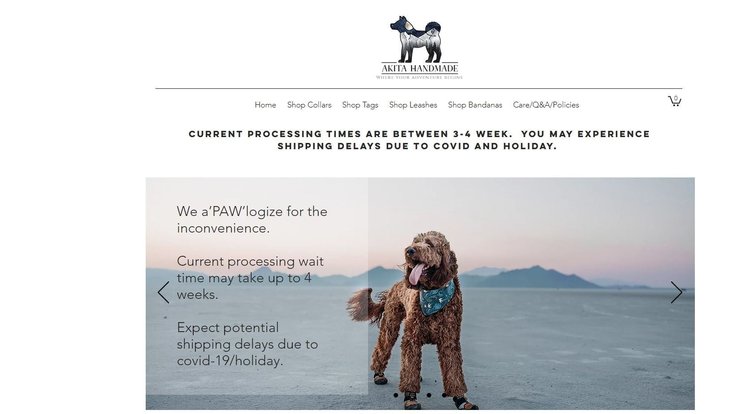The top section of the image displays the following text: "Akita Handmade" with a line beneath it, followed by "Home," "Shop Collars," "Shop Tags," "Shop Leashes," "Shop Bandanas," "Care," "Q&A," and "Policies." Below this, a notice reads, "Current Processing Times are between 3-4 weeks. You may experience shipping delays due to COVID and a holiday."

Below this header is a picturesque scene featuring a dog with curly hair trotting through the snow. The dog is adorned with a blue bandana around its neck. The backdrop consists of snow-covered terrain, flat expanses of land, and majestic mountains under a purplish sky, possibly suggesting a location near the North Pole.

On the left side of the image, there is a noticeable box that reads, "We P-A-W-L-O-G-I-Z-E for the Inconvenience." The box continues with the message, "Current Processing Wait Time may take up to 4 weeks. Expect potential shipping delays due to COVID-19/holiday." The remainder of the image is largely composed of white, empty space.